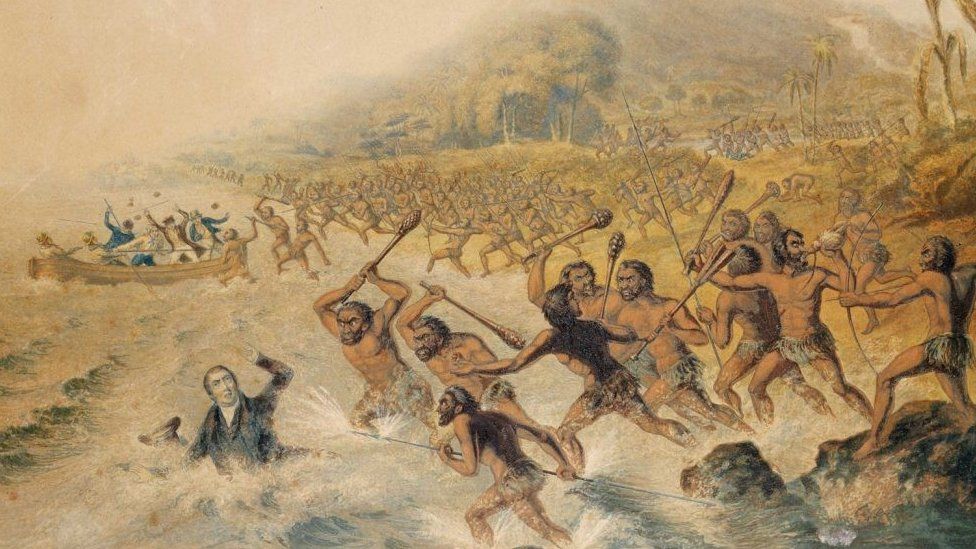In this detailed, old-style color illustration, we witness a dramatic and chaotic battle scene unfolding on a beach. Dominating the foreground is a lighter-skinned man standing in the water, dressed in a suit with his hat floating nearby. His expression of despair is stark as he raises his left arm in a defensive gesture. Charging towards him from the beach are numerous indigenous people wielding clubs and spears, bare-chested and clad in loincloths, poised to strike. This mass of native warriors, emphasizing their overwhelming numbers, cascades down the beach and into the water, creating a sense of imminent danger.

On the left side of the painting, several men are arriving on a boat, dressed in colonial-style clothing. These well-dressed men, seemingly outnumbered and frightened, are readying themselves for combat. Further back on the left, more boats can be seen, hinting at additional reinforcements or fleeing colonists.

In the background, beyond the beach, trees and a hill emerge, gradually fading into a plain white canvas, which adds depth to the chaotic scene. On the far right, one man stands on a rock, pulling back a bow and arrow, ready to shoot. Nearby, another man blows a horn, signaling to others amidst the turmoil. The entire scene conveys a vivid and detailed struggle between the indigenous warriors and the invading colonial forces, filled with tension and imminent violence.